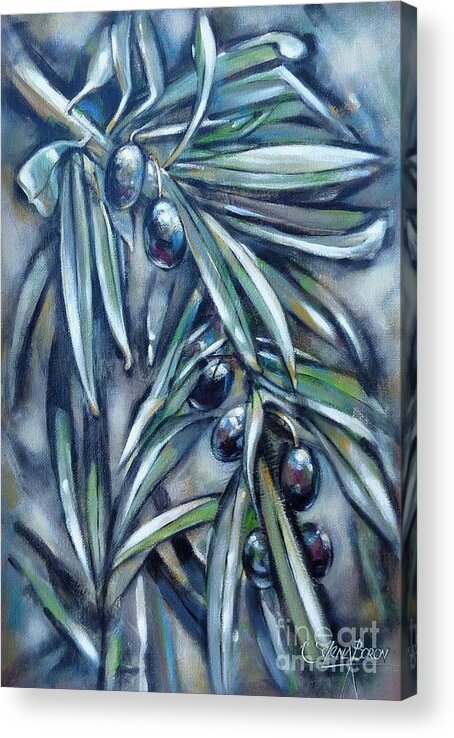The photograph showcases a dramatic 3D-style canvas painting that appears to pop off the wall due to its frame extending an inch or two outward. The painting, set against a white wall, features an olive branch with black olives and intricate leaves. In the top left corner of the painting, a branch adorned with thin, long leaves and two black olives is prominently displayed. The bottom right corner reveals another branch supporting a cluster of five black olives. The background is an abstract mix of greens, whites, and blacks that accentuates the depth around the olive branches, creating a striking contrast and sense of dimension. The color palette is predominantly monochrome, focusing on shades of blue, green, and black, with dramatic contouring and highlights enhancing the three-dimensional effect. A semi-transparent watermark at the bottom right, reading "Fine Art America," slightly obscures a signature, adding a final touch to this detailed and textured piece of art.